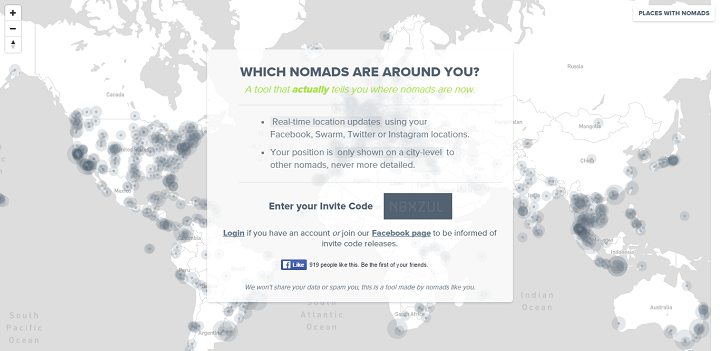The screenshot depicts a map interface, likely viewed on a desktop, showcasing a grayscale world map. The map features dark gray oceans and white continents, with North America and South America positioned on the left side of the screen, Greenland at the top, Africa and Europe centrally located, and Asia, Southeast Asia, and Australia on the right.

Scattered across the map are circles in varying shades of gray, each punctuated by a black dot representing locations and the number of people in each area. Key regions with notable activity include the United States, South America, Europe, and Southeast Asia.

At the center of the screen, there is a light gray transparent box with black text that reads, "Which nomads are around you," followed by green text explaining a tool that indicates the current locations of nomads. Below are bullet points detailing the features of this tool:
- "Real-time location updates using your Facebook, Swarm, Twitter, or Instagram."
- "Your position is only shown at a city level to other nomads, never more detailed."

Additionally, the box prompts users to "Enter your invite code," displaying an unreadable gray box meant for the code entry, followed by options to "Log in if you have an account" or "Join with our Facebook page to be informed of invite code releases." A Facebook like icon is also present at the end.